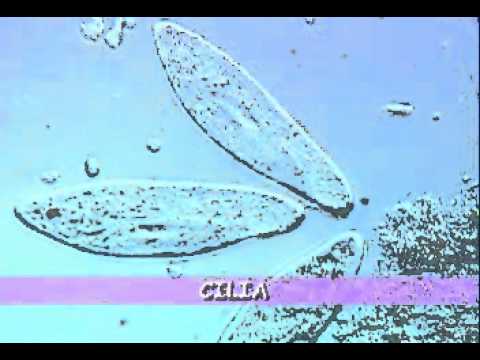The image appears to be a blurry microscopic view, characterized by a black border on the top and bottom, suggesting it could be a still from a movie or PowerPoint presentation. The background is a light blue or turquoise, showing several clear, banana-shaped or elliptical structures outlined in black. Among these large elliptical shapes, which are spread across the image, there are numerous small black specks and circles clumped together, with a particularly large cluster in the lower right corner. Additionally, there is a significant irregular structure on the bottom left, filled with many black spots. A prominent purple ribbon is displayed horizontally near the bottom of the image, with the word "Cilia" written in white Comic Sans font, indicating that the image likely depicts cilia – tiny hair-like structures found within the human body, typically observed under a microscope.